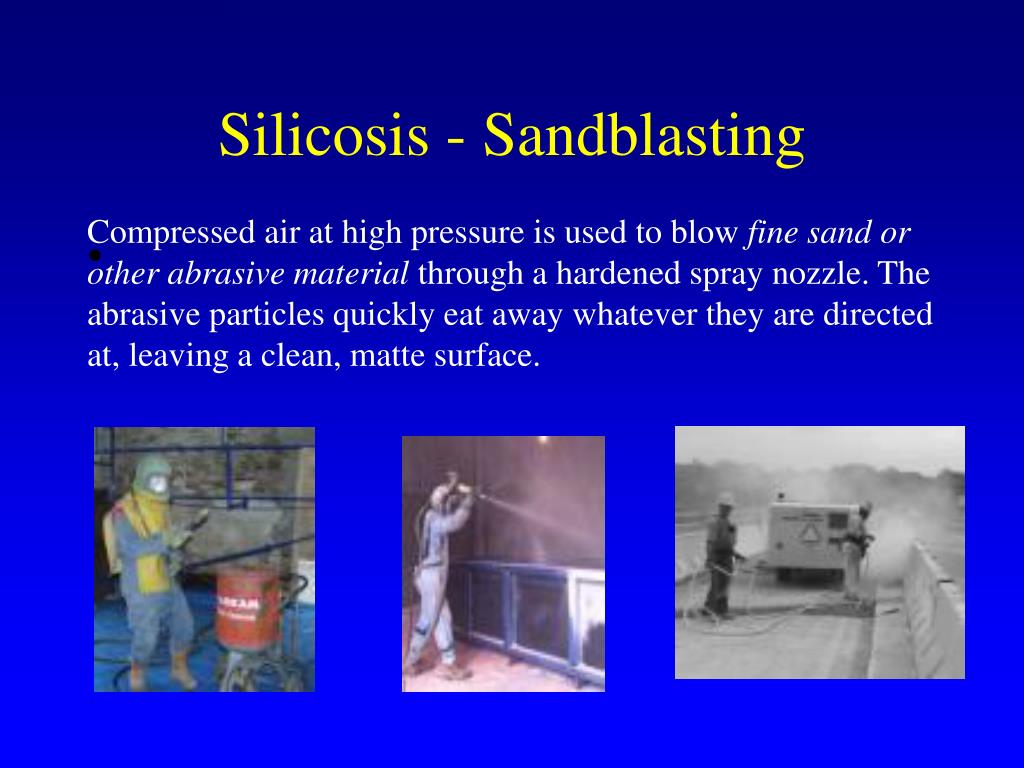The PowerPoint slide features a blue background that transitions from a lighter hue at the bottom to a darker shade at the top. The prominent headline, "Silicosis - Sandblasting," is displayed in vibrant yellow text. Beneath the headline, the accompanying white text reads: "Compressed air at high pressure is used to blow fine sand or other abrasive material through a hardened spray nozzle. The abrasive particles quickly eat away whatever they are directed at, leaving a clean, matte surface."

Below this informative text, three photographs are arranged horizontally. The leftmost image shows a worker clad in a blue hazmat suit with a yellow vest, donning a green helmet. He is holding a sandblasting device, and next to him stands a large, red cylinder, suggesting an industrial environment. The middle photograph depicts another worker in a full-body protective light gray suit, actively spraying a substance downward, likely engaged in sandblasting a metal fence. The rightmost photograph, presented in black and white, captures two men on a concrete bridge. They are operating a sandblasting machine connected to a pipe from a truck, focused on cleaning the jersey barriers.